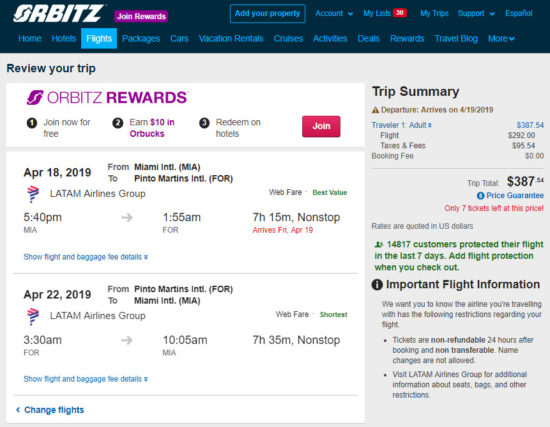The image appears slightly blurry, but several key elements are identifiable. 

In the top-left corner, there's a white "ORBITZ" logo. Right underneath it, a pink tab says "Join Rewards." Below the logo is a navigation bar with various blue-colored tabs: Home, Hotel, Flight (highlighted in blue), Packages, Cars, Vacation Rentals, Cruises, Activities, Deals, Rewards, Travel Blog, and More. 

Above the navigation bar, on a dark blue background, there are additional links written in blue: Español, Support, My Trips, My List (highlighted in red), Account, and "Add Your Property." 

Within the light gray background area below the header, the left side reads "Review Your Trip" in dark blue text. There’s also a pink "ORBITZ Rewards" banner with steps: 
1. Join now for free.
2. Earn $10 in Orbucks.
3. Redeem on hotels.
Next to this, a prominent red "Join" button appears.

Further down, detailed flight information is provided for a departure on April 18, 2019, with LATAM Airlines Group from Miami International to Pinto Martins. The flight leaves at 5:40 p.m. and arrives at 1:55 a.m., with a duration of 7 hours and 15 minutes, labeled as "Webfare Best Value" in red, arriving on Friday, April 19.

The right side features a "Trip Summary" section, indicating a departure on April 19, 2019, in brown text. The summary includes:
- Traveler: One adult
- Price: $387.59
- Flight: $292.00
- Taxes and Fees: $94.54
- Booking Fees: $0.00
- Total: $387.54

Highlighted in red is a note that only seven tickets are left at this price, and the rates are quoted in US dollars. A green text mentions that 14,817 customers protected their flights in the last seven days, with an option to "Add Flight Protection" during checkout.

Finally, there's an "Important Flight Information" section, detailing that the airline's restrictions, such as tickets being non-refundable, can be reviewed on LATAM Airlines Group's website.